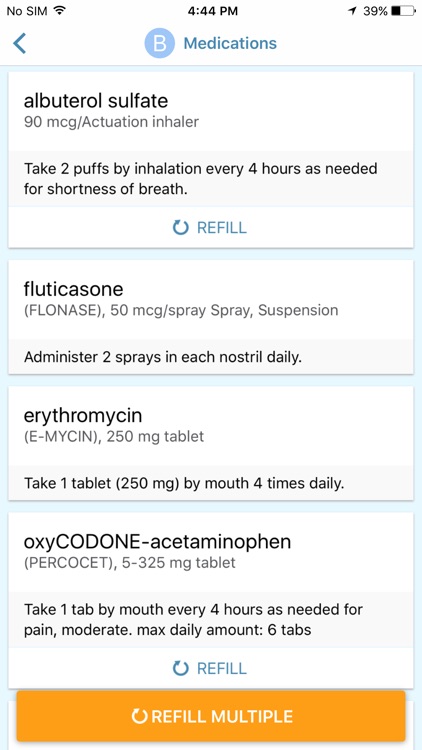### Detailed Caption:

The image appears to be a screenshot taken from a smartphone displaying a medication management application on a computer screen. At the top of the screen, there is a header labeled "Medications," accompanied by a capital letter 'B' inside a periwinkle-colored circle, with the letter 'B' displayed in white. To the left of the header is a left-pointing arrow.

In the upper-left corner of the screen, the status bar indicates "No Sim" and the current time as 4:44 p.m. The battery icon shows a 39% charge, depicted graphically with a mostly white battery containing a black segment to represent the remaining power.

The medication list begins with "Albuterol Sulfate 90 MCG Activation Inhaler," which instructs the user to "take two puffs by inhalation every four hours as needed for shortness of breath." Beneath this instruction is a clickable refill option, designated by a rotating arrow and the word "REFILL" written in blue, uppercase letters.

Following the Albuterol entry is a list of other medications:
1. "Fluticasone Propionate 50 MCG (Flonase) Spray Suspension," with the instruction to "administer two sprays in each nostril daily."
2. "Erythromycin" and "Oxycodone."

At the bottom of the screen, there is an orange button labeled "Refill Multiple," allowing the user to manage multiple medication refills efficiently.

The interface is clean and user-friendly, designed to help individuals manage their prescriptions seamlessly.